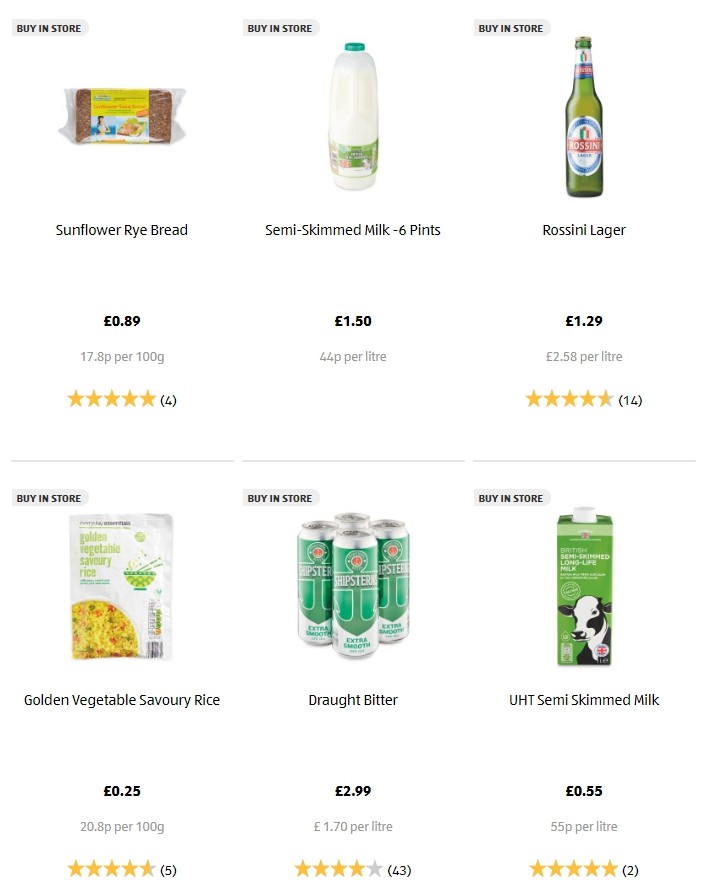The image displays a section of a pick-and-save app interface featuring six different grocery items available for selection and purchase. From left to right, the items displayed are:

1. **Sunflower Rye Bread** – Available for in-store purchase or delivery, this bread is prominently marked for easy identification.
2. **Semi-Skimmed Milk (Six Pints)** – Priced at £1.50, this milk option provides an economical choice for buyers.
3. **Rossini Lager** – A beer option, possibly appealing to those looking for alcoholic beverages.
4. **Golden Vegetable Savory Rice** – A convenient and tasty side dish for home-cooked meals.
5. **Draft Bitter** – Another beer choice, catering to different tastes in alcoholic beverages.
6. **Semi-Skimmed Milk** – Another listing of semi-skimmed milk, indicating its popularity and necessity.

Pricing for each item is clearly listed in British pounds, suggesting the app is UK-based. Detailed product stars and review ratings accompany five of the six items, giving users insight into consumer satisfaction, with one item lacking any reviews. Information about price per liter or specific measurement per container/package is also provided, aiding users in making informed purchasing decisions.